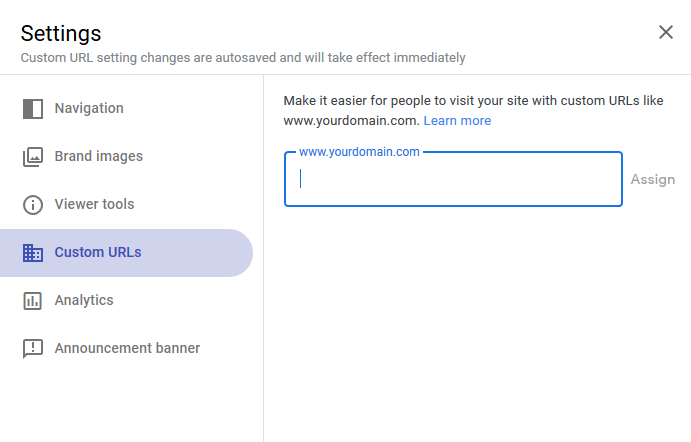The image displays a settings section on a computer interface, identifiable by the prominent "Settings" label in black located at the upper left-hand corner. Most of the other text is in gray. Directly below this label, it states, "Custom URL setting changes are auto-saved and will take effect immediately," followed by a straight horizontal line dividing the section.

Under this line, there is a vertically aligned menu of different settings categories, each with accompanying icons. The categories listed from top to bottom are:
1. Navigation
2. Brand Images
3. Viewer Tools
4. Custom URLs (which is highlighted)
5. Analytics
6. Announcement Banner

On the right-hand side of the image, a vertical line is drawn about a third of the way from the left, providing a clear separation. Within this right section, there is a message in gray text urging users to facilitate site visits with custom URLs, such as "www.yourdomain.com." Below this message, a clickable "Learn More" link appears in light blue.

Beneath the informational text, there is a horizontal blue rectangle containing the placeholder text "www.yourdomain.com" on the left side. Adjacent to this blue rectangle on the right side is a button labeled "Assign."